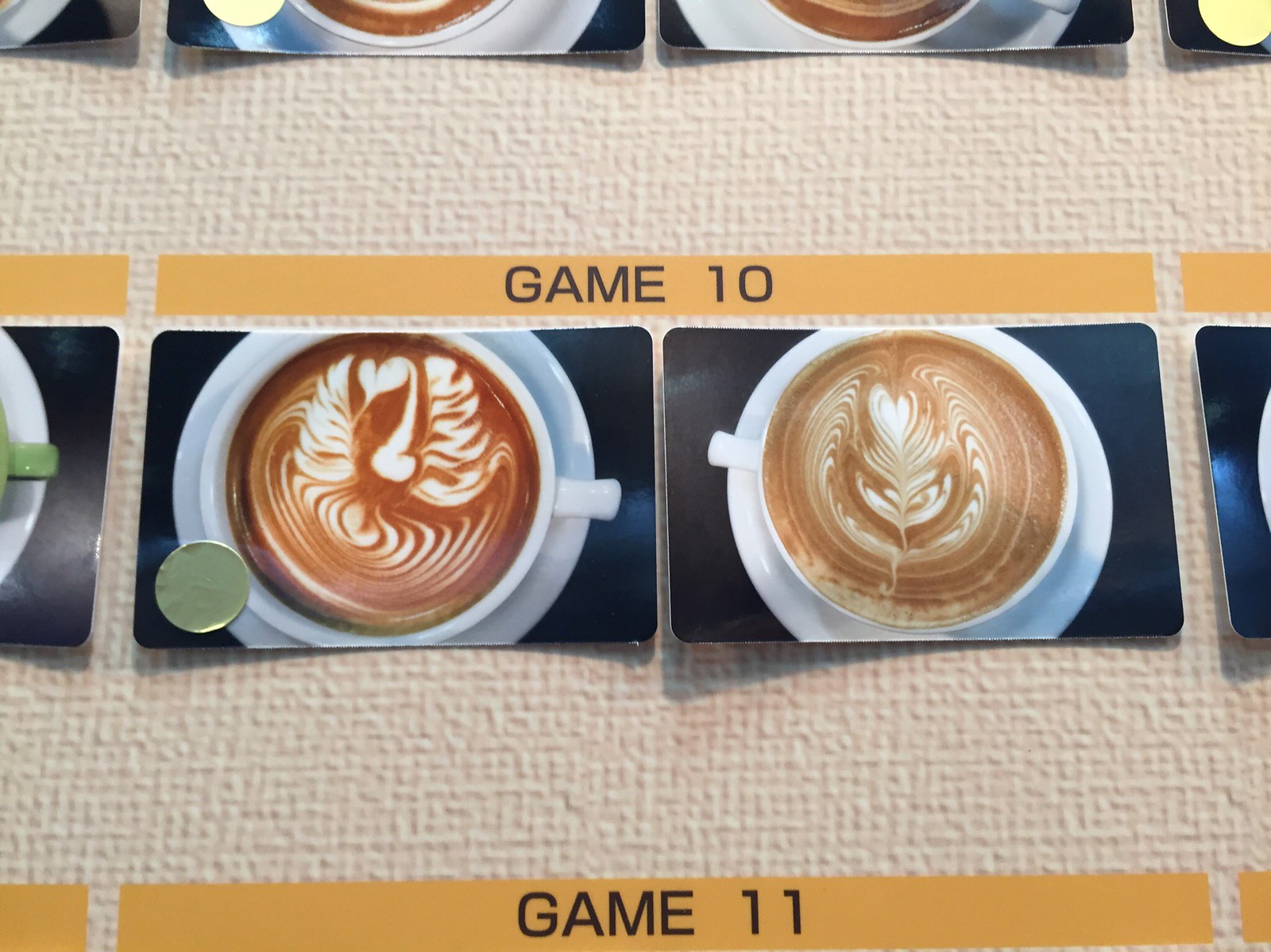In the image, there are photographs of various food items, predominantly featuring cups of cappuccino or latte with intricate cream designs. The background is a patchy light salmon beige, with orange bars across the middle and bottom containing black text. On the top bar, written in all capitals, is "GAME 10," and on the lower bar is "GAME 11," both text strips being yellow in color. Below the "GAME 10" bar, there are two top-down photographs of cappuccinos. The cup on the left contains a darker brown coffee in a white cup on a white saucer, adorned with a squiggly line cream design and a green sticker in the bottom left corner. The cup on the right contains a lighter brown coffee in a similar white cup and saucer, with a cream pattern resembling a flower. These coffee photographs are laid out in a row atop what appears to be a textured, off-white sheet.